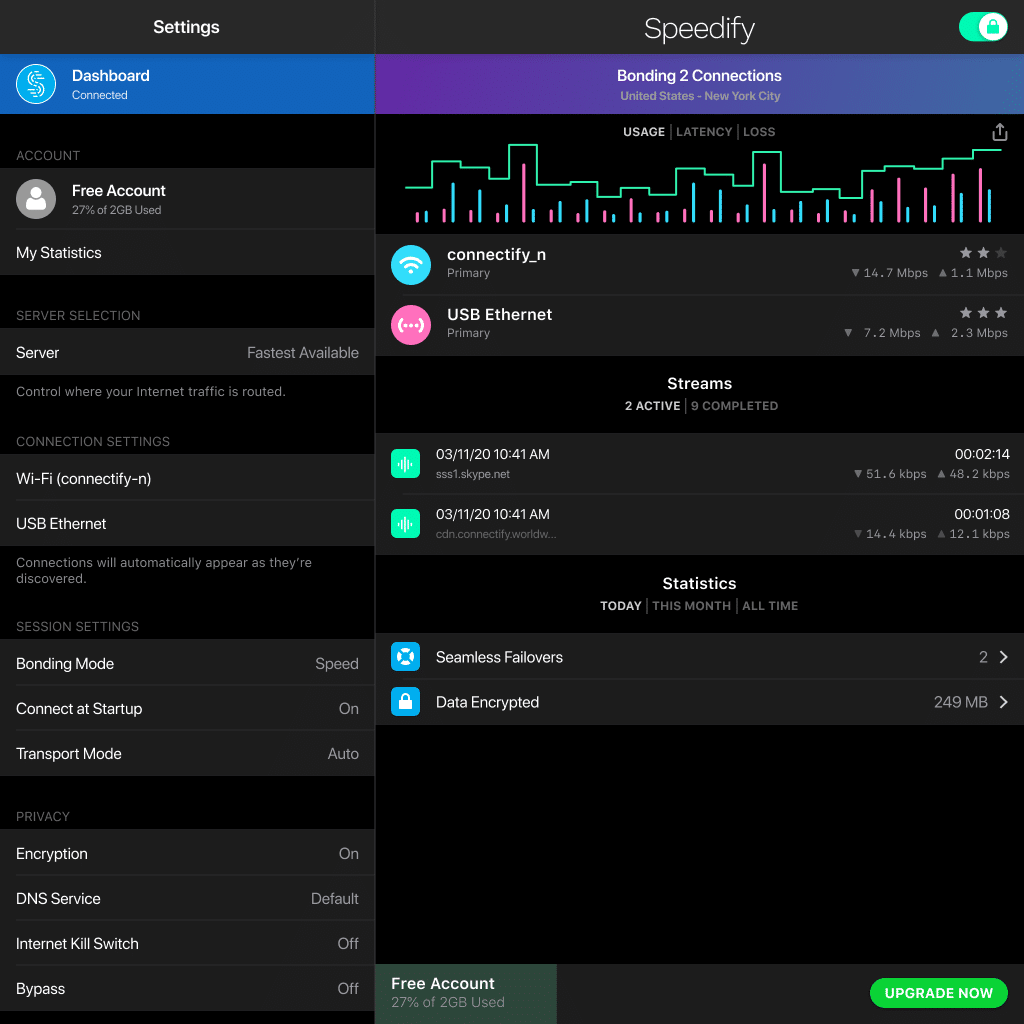In the image, we see an interface for the Speedify application, specifically a page designed to monitor connections. The layout includes several key elements such as settings, a dashboard, and options for connection bonding. The application interface shows a user with a free account, indicating that 27% of their 2GB data limit has been used. 

Highlighted on the page are various sections, including "My Statistics," "Server," "Fastest Available," "WiFi," "Connectify," and "USB Ethernet." The connections are set to automatically appear as they are discovered. Additionally, the interface displays several configuration settings: bonding mode, speed, "Connect at Startup" enabled, transport mode set to automatic, encryption enabled, DNS service set to default, internet kill switch turned off, and bypass disabled.

The connection details reveal that the primary connection through "Connectify" is operating at a speed of 14.7 Mbps, while the secondary "USB Ethernet" connection is running at 7.2 Mbps. The color palette of the image comprises shades of blue, purple, white, and pink, set against a black background, providing a visually appealing contrast that helps in distinguishing various elements on the interface.